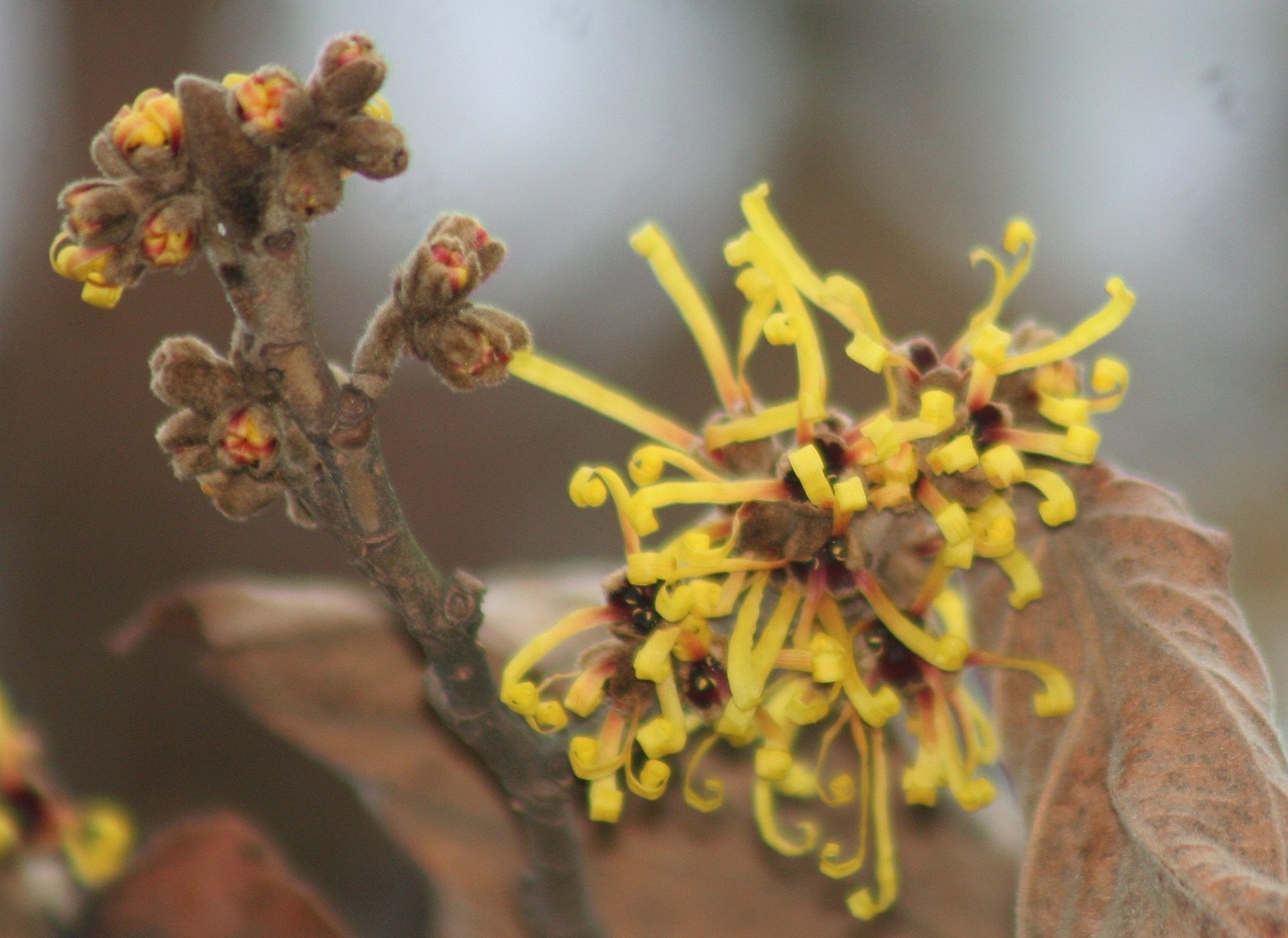In the foreground of the image, a single plant draws attention, showcasing both budding and mature flowers in striking contrast. To the left, the plant features a stem with budding yellow and red flowers, poised to bloom. On the right, the mature flowers display long, stringy petals in shades of red and yellow, curling at the ends. Adjacent to these mature flowers, a browning or dead leaf suggests the cycle of life and decay. The central flower, which appears to be in the process of dying, anchors the composition of the image. The background is completely blurred out, emphasizing the plant and creating a sense of isolation.